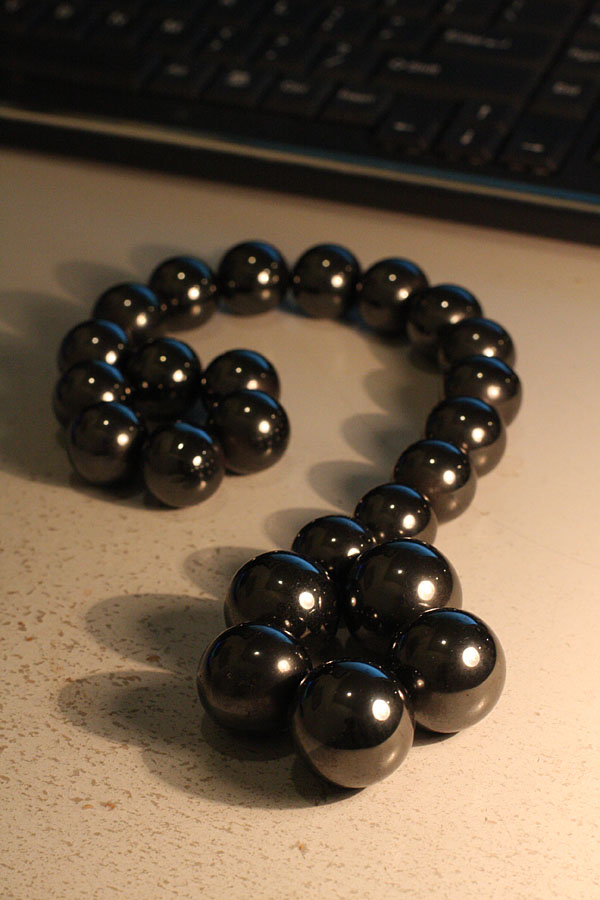A detailed indoor photograph captures a striking arrangement of natural black magnetic hematite orbs, each approximately 15 millimeters in diameter, laid out on an off-white cream-colored desk surface with chipping paint revealing a tan undertone. The orbs, forming a question mark shape with both ends curling into spirals, taper in size with the largest spheres at the ends. The light source from the lower right creates a reflective white dot on the glossy surface of each sphere. In the blurred background, a black keyboard can be seen, emphasizing the focused detail of the orbs in the foreground. The overall setup suggests they could be part of a necklace, though it's unclear if they are strung together or simply arranged in this form.